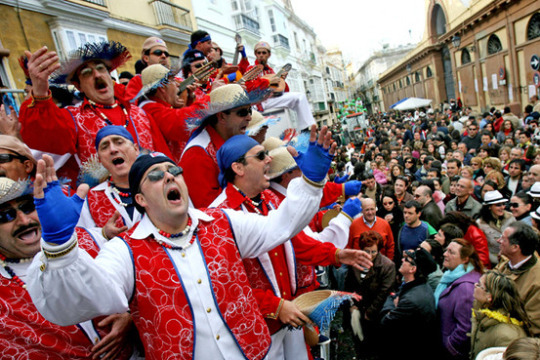The image depicts a vibrant, festive scene, likely a parade or street fair, held in a densely crowded street flanked by tightly packed, multi-story buildings in various shades of brown, yellow, and white. On the left side of the frame, a group of men stands out with their distinctive attire: white shirts, red vests speckled with blue bubbles, white pants, and blue fingerless gloves. These men, some adorned with blue head wraps, straw hats, baseball caps, and beads around their necks, appear to be entertainers, possibly a mariachi band, as they sing and raise their arms, engaging the crowd. A couple of stringed musical instruments can be seen in the background, adding to the lively atmosphere. The dense crowd, full of spectators in jackets and hats, stretches across the street, giving a sense of the immense turnout. A tractor and other elements are visible behind the entertainers, contributing to the bustling, happy ambiance of the scene. The sky overhead is a bright white, casting an even, diffuse light over the festive gathering.